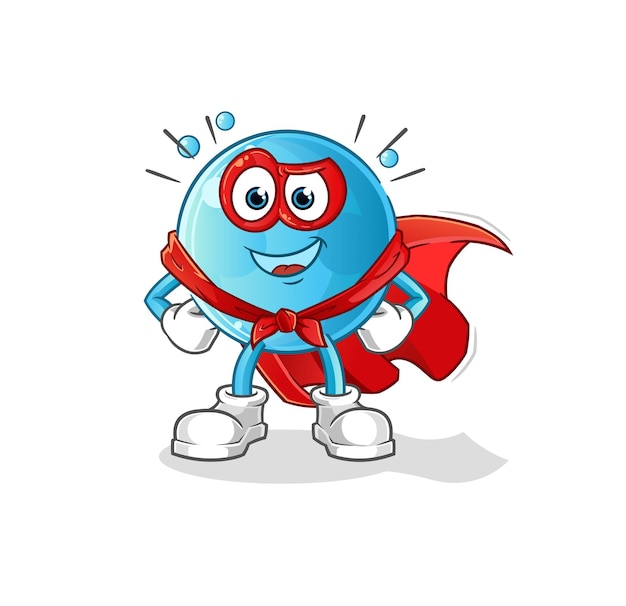The image depicts a cartoon-style superhero characterized by its round, gumball-like blue body. The character stands on thin blue legs with white boots and has thin blue arms adorned with white gloves, which are positioned on its hips. It features a red mask around its large oval white eyes, detailed with blue irises and black pupils. The mouth is open in a happy expression, revealing a maroon-red tongue. On its head, there are three small blue bubbles and three black lines sticking out on either side, adding to its lively appearance. The character also dons a red cape, tied around its front and billowing behind, suggesting action or movement.